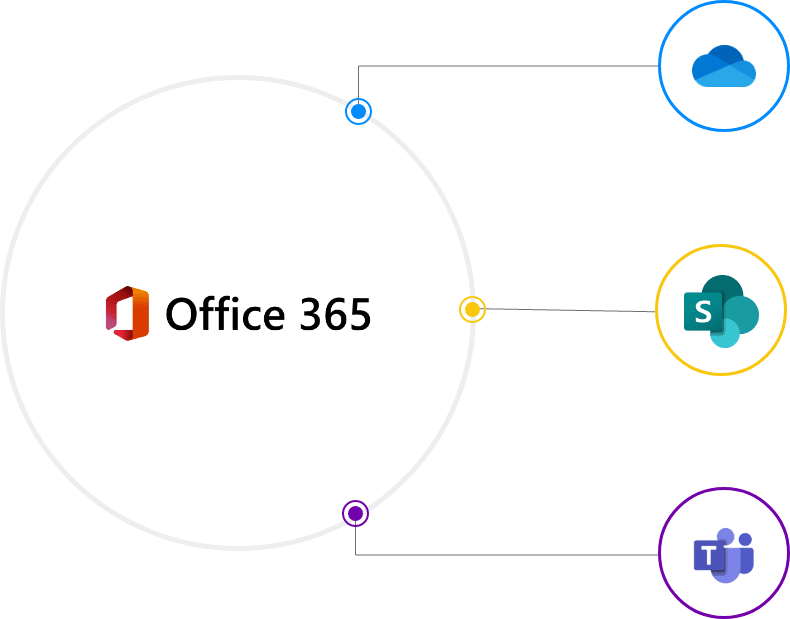This screenshot showcases a detailed chart illustrating the relationships and integrations within Office 365. Positioned at the left of the chart, within a light gray circle, is the red Office 365 logo. Moving directly to the right, this gray circle extends to a series of interconnected elements.

The first element encountered is a yellow dot encased in a yellow circle, from which a gray line extends further to the right. This line connects to another yellow circle, housing an icon featuring an 'S' inside a green box. Surrounding this green box, there are three layered circles of varying shades: a dark green circle, a teal circle, and a smaller light teal circle.

Beneath this structure is another purple circle encircling a box with a 'T' inside. Adjacent to this is a violet person icon layered over another purple person icon. Extending from these elements, a gray line arcs back to the original circle and then upwards, leading to another purple circle.

Directly above, a blue circle emerges, prominently featuring the blue OneDrive logo. This composition reveals three main colored circles—yellow, purple, and blue—situated on the right side of the image. Each of these circles and their respective connections originate from the central Office 365 logo, illustrating the cohesive and integrated nature of the Office 365 suite.